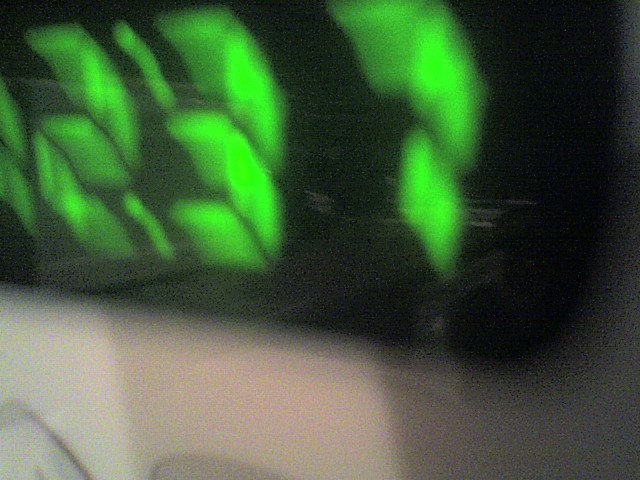The image captures an up-close, blurry view of a black digital alarm clock with lime green numbers displaying the time 12:37. The photo is heavily blurred, likely due to camera movement, causing the colors to smear across the clock's black screen, which also appears slightly reflective. The clock is sitting on a beige or white shiny surface that resembles a typical end table or nightstand from the 80s. The background features a light beige surface, and there's an indistinct shadow or possible wall edge to the right side of the clock. The green digital numerals are strikingly fluorescent, akin to an alien green hue, adding to the image's nostalgic and somewhat surreal appearance.